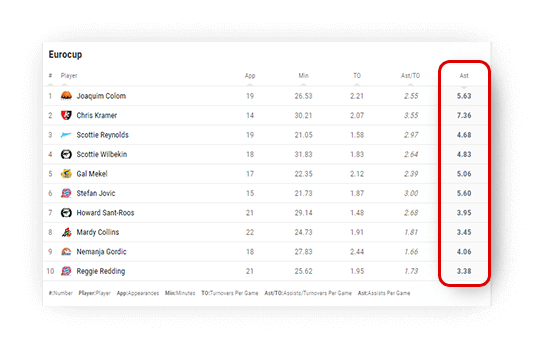This image showcases a detailed list of sports statistics for various players participating in the Euro Cup. In the top left corner, there's the Euro Cup logo. The table is structured with vertical lines creating separate columns. There are 10 entries, each numbered from 1 to 10. 

To the right of the numbers, small icons accompany the players' names, which are as follows: 
1. Joaquin
2. Colum
3. Chris Kramer
4. Scotty Reynolds
5. Scotty Wilkins
6. Gail McGill
7. Stefan Joyce
8. Howard Stantruse
9. Marty Collins
10. Nemanja Gordic
11. Reggie Redding

Further to the right, there are columns titled "APP" (possibly appearances), "MIN" (likely minutes), "TD" (possibly touchdowns), and "Assisted TDs" to systematically present player statistics. The final column on the right has text that is too small to read clearly.